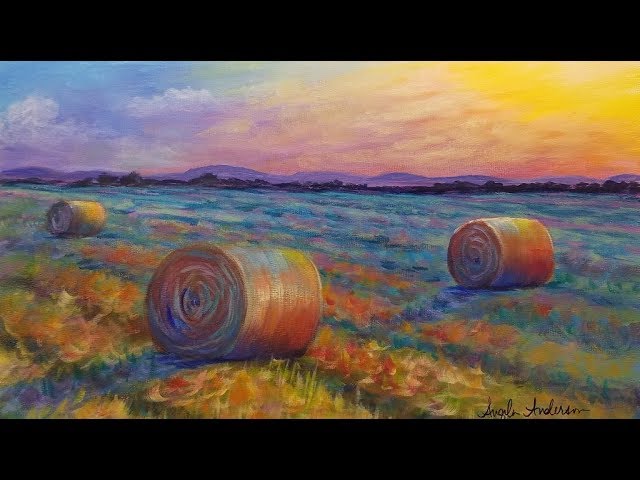The painting depicts a harvested hay field under a vibrant sunset. In the foreground, three large, rolled hay bales rest on the short-cut grass, casting long shadows. The field transitions from rich yellows to cooler blues as it stretches into the distance, framed by a distant line of trees and low mountains. The sky above is a dynamic blend of colors, with shades of yellow, red, blue, purple, and pink, capturing the essence of the setting sun. The artwork is signed in cursive at the bottom right, likely by Angela Anderson, with black bars framing the top and bottom of the painting.